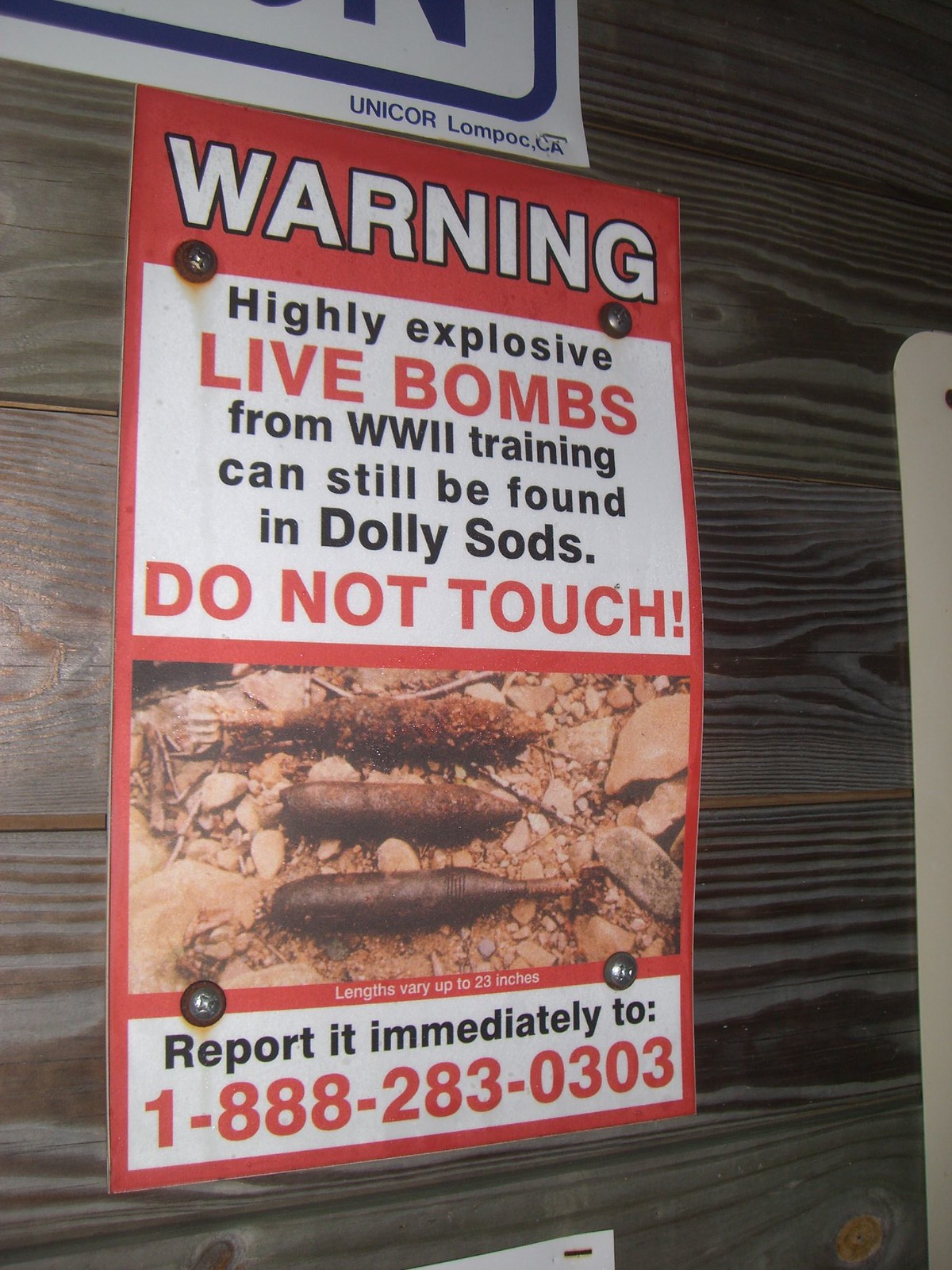This image depicts a warning poster affixed to a wooden wall, cautioning the public about the presence of live bombs from World War II training exercises that can still be found in Dolly Sods. The poster prominently features the text: "Warning: Highly explosive bombs from World War II training can still be found in Dolly Sods. Do not touch. Report immediately to 1-888-283-0303." The text varies in color, with white, red, and black lettering used to emphasize different parts of the warning. The poster also includes rusted images of the World War II bombs, which are cylindrical in shape, approximately three inches in height and one inch thick, and are depicted lying side by side on a rocky, dirt-strewn ground amidst small branches. The setting suggests an outdoor environment, possibly on the side of a wooden building, cluttered with various other posters and papers.